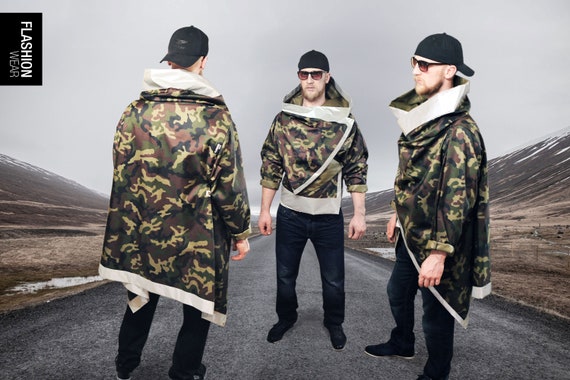In this detailed photograph, three identical representations of the same man are positioned on an asphalt road against a backdrop of brown, snow-capped mountains under a light gray sky. Each man is outfitted in a matching camouflage jacket with a cape-like back, and they wear baseball caps turned backward, dark sunglasses, black pants, and identical footwear. The central figure faces the camera, revealing a small scruffy beard and rolled-up sleeves, while the figures to the left and right display side and back angles, respectively, showcasing different views of the jacket. A black square in the top left corner bears the text "fashion wear" in vertical letters, with "fashion" in a lighter shade and "wear" in light gray. These portraits appear designed to highlight the versatility and comprehensive view of the apparel from various perspectives.